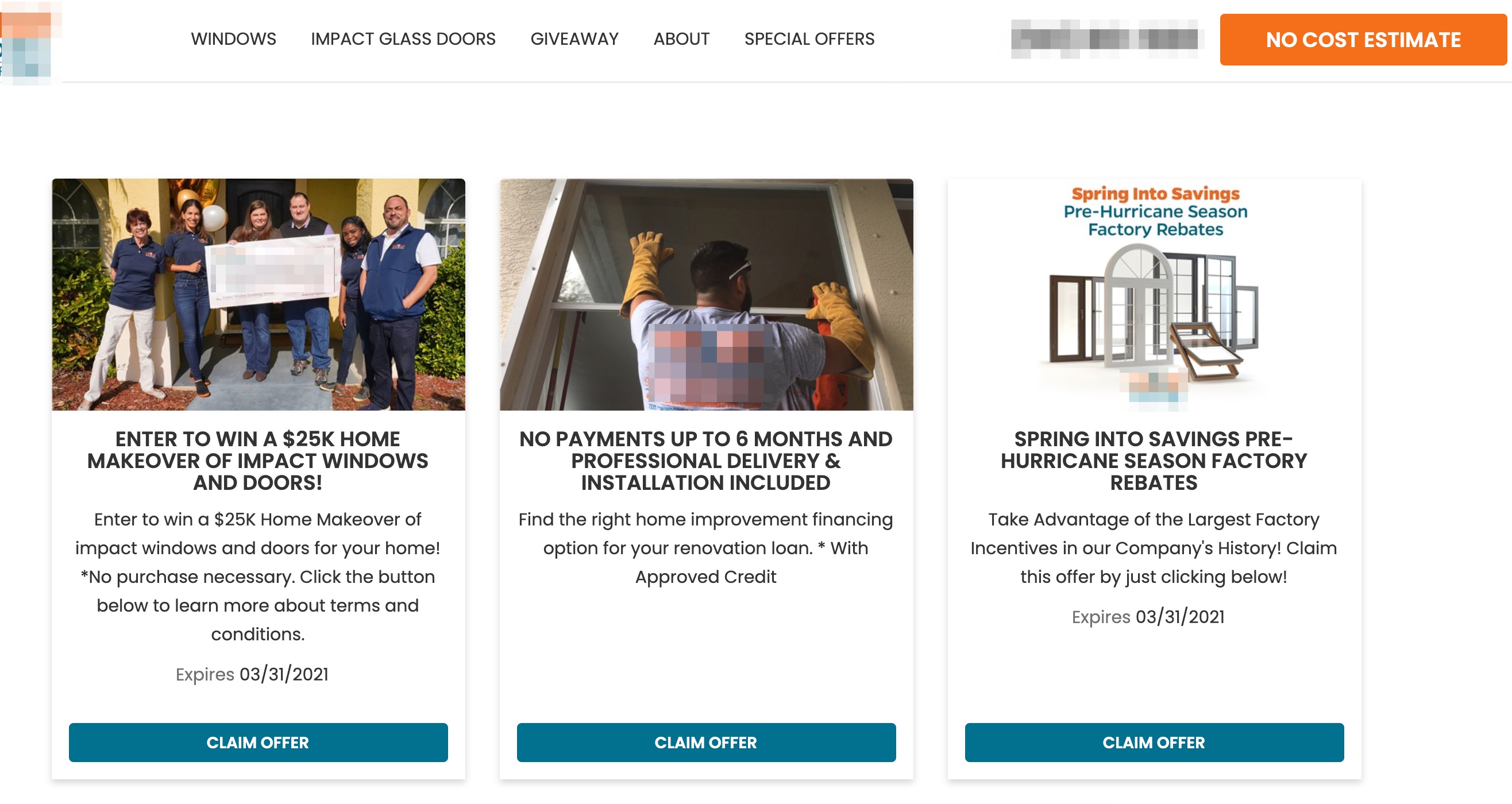Screenshot of a promotional webpage for a home improvement giveaway. The webpage features a pixelated and grayed-out logo with a yellow, blue, and white banner. At the top of the white background, we see navigation links labeled "Windows," "Impact Glass Doors," "Giveaway," "About," and "Special Offers" in a black font. 

A partially grayed-out section follows, next to which is an orange button labeled "No Cost Estimate." Below is an image of smiling people standing in front of a home, holding a large check. The text on the check reads, "Enter to win a $25,000 home makeover of impact windows and doors." 

Adjacent to this image is a blue "Claim Offer" button, with a note stating, "Expires 3-31-2021." The promotion details that there is no purchase necessary and prompts visitors to "click the button below to learn about terms and conditions." 

The middle section of the page includes a photograph showing a person installing windows. The accompanying text reads, "No payments up to six months," and mentions that professional delivery and installation are included. Another call-to-action for "Claim Offer" and mentions "Spring into Savings pre-hurricane season factory rebates."